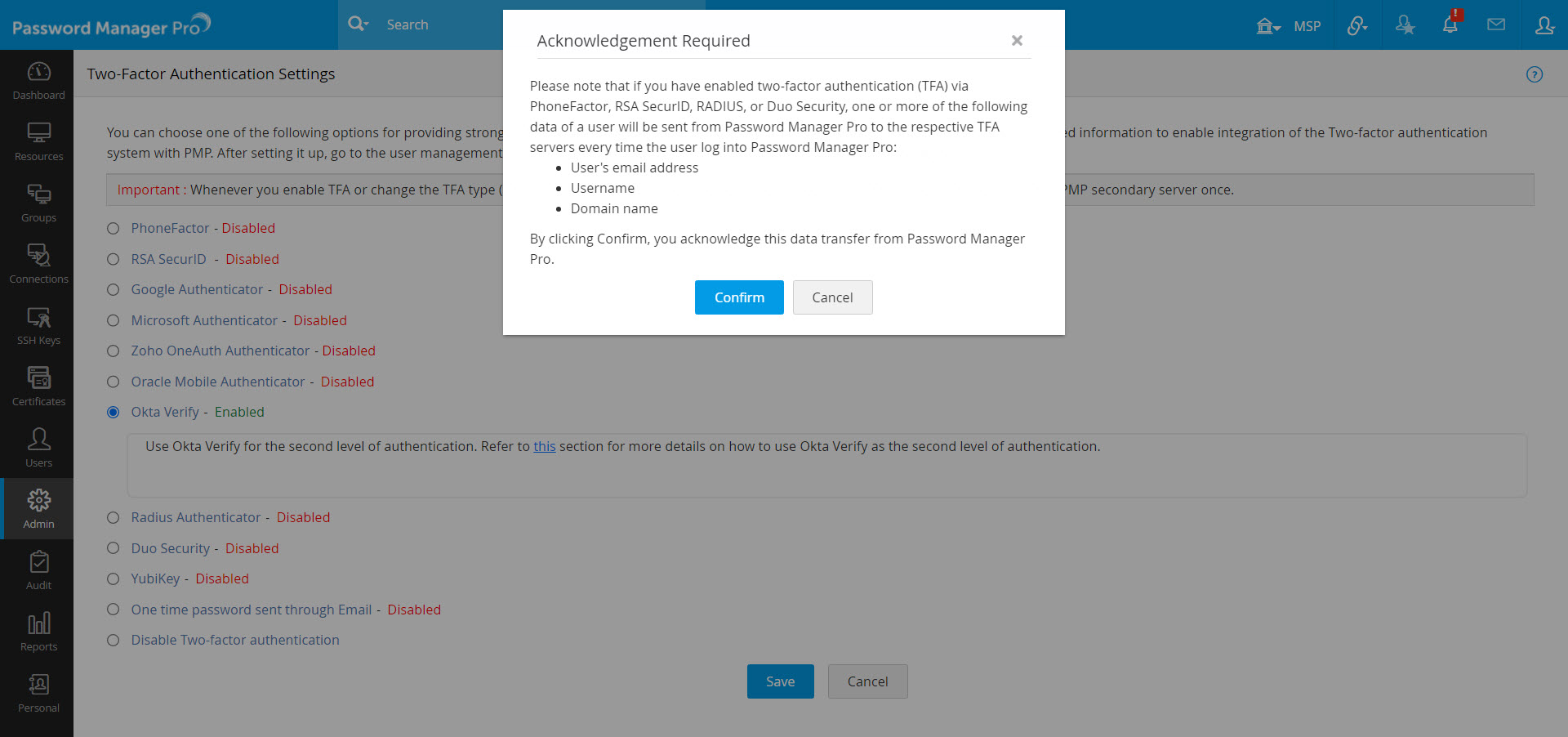Screenshot of a Password Manager Interface with Two-Factor Authentication Prompt

The screenshot features the user interface of a password management application called "Password Manager Pro," as indicated by the title in the top left corner. Prominently displayed in the center is a pop-up window titled "Acknowledgement Required." This pop-up message informs the user about data transmissions related to enabling two-factor authentication (TFA). Specifically, the pop-up explains that if TFA methods such as Phone Factor, RSA SecureID, RADIUS, or Duo Security are activated, certain user data—including email address, username, and domain name—will be sent to the designated TFA servers each time the user logs in. To acknowledge this data transfer, the user must click "Confirm" at the bottom left of the pop-up window, or they can cancel by clicking "Cancel" at the bottom right.

In the background, it is evident that multiple TFA options have been disabled, leaving OKTA Verify as the only active method. A message highlights that OKTA Verify is being used for the second level of authentication and provides instructions for more details on utilizing OKTA Verify effectively.